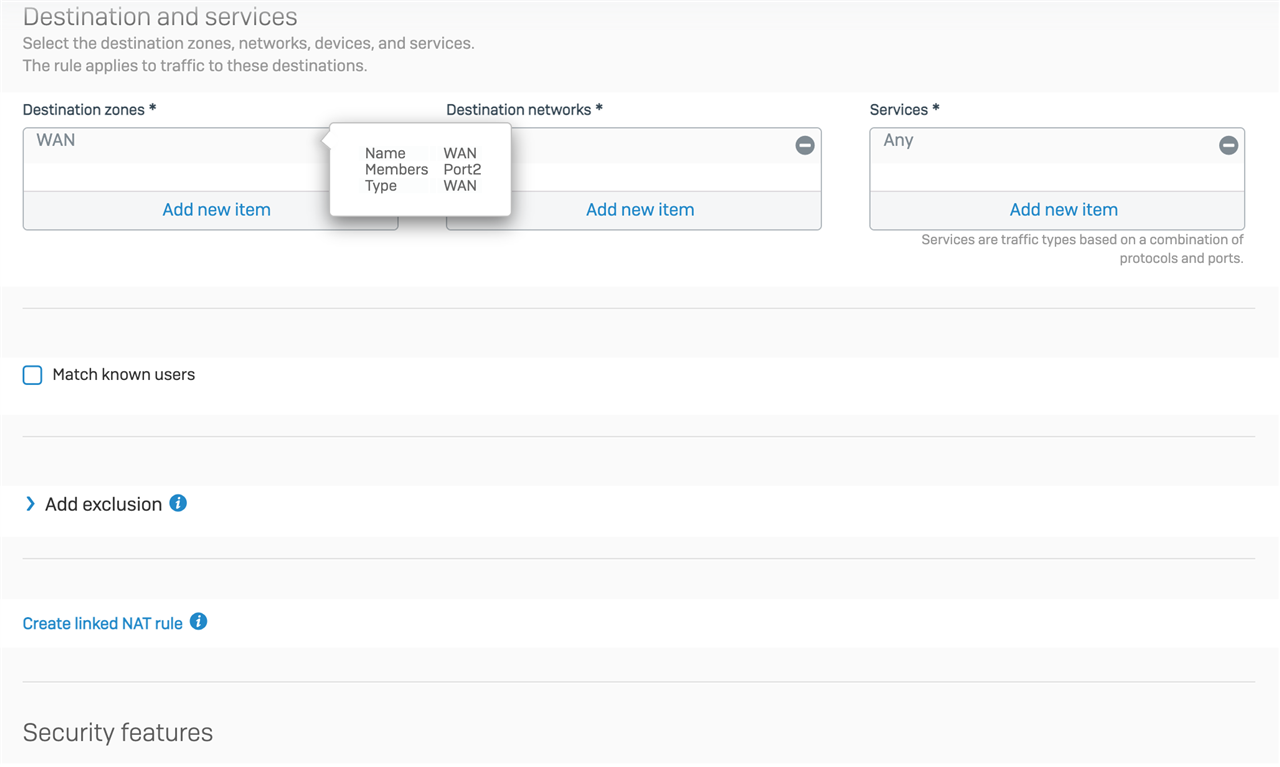A detailed description showing the configuration interface of a network security system:

"Screenshot of a network security system's configuration interface, illustrating the process of setting up destination rules for restricted traffic. The interface allows users to select specific destination zones, such as WAN. The user has added 'WAN' as the destination zone and labeled it 'port 2'. The interface also shows options to add new destination networks and services. In this instance, 'any' service and any traffic type based on various combinations of protocols and ports are selected. Additional features include options to match known users, add exclusions, and create linked NAT (Network Address Translation) rules for enhanced security measures."